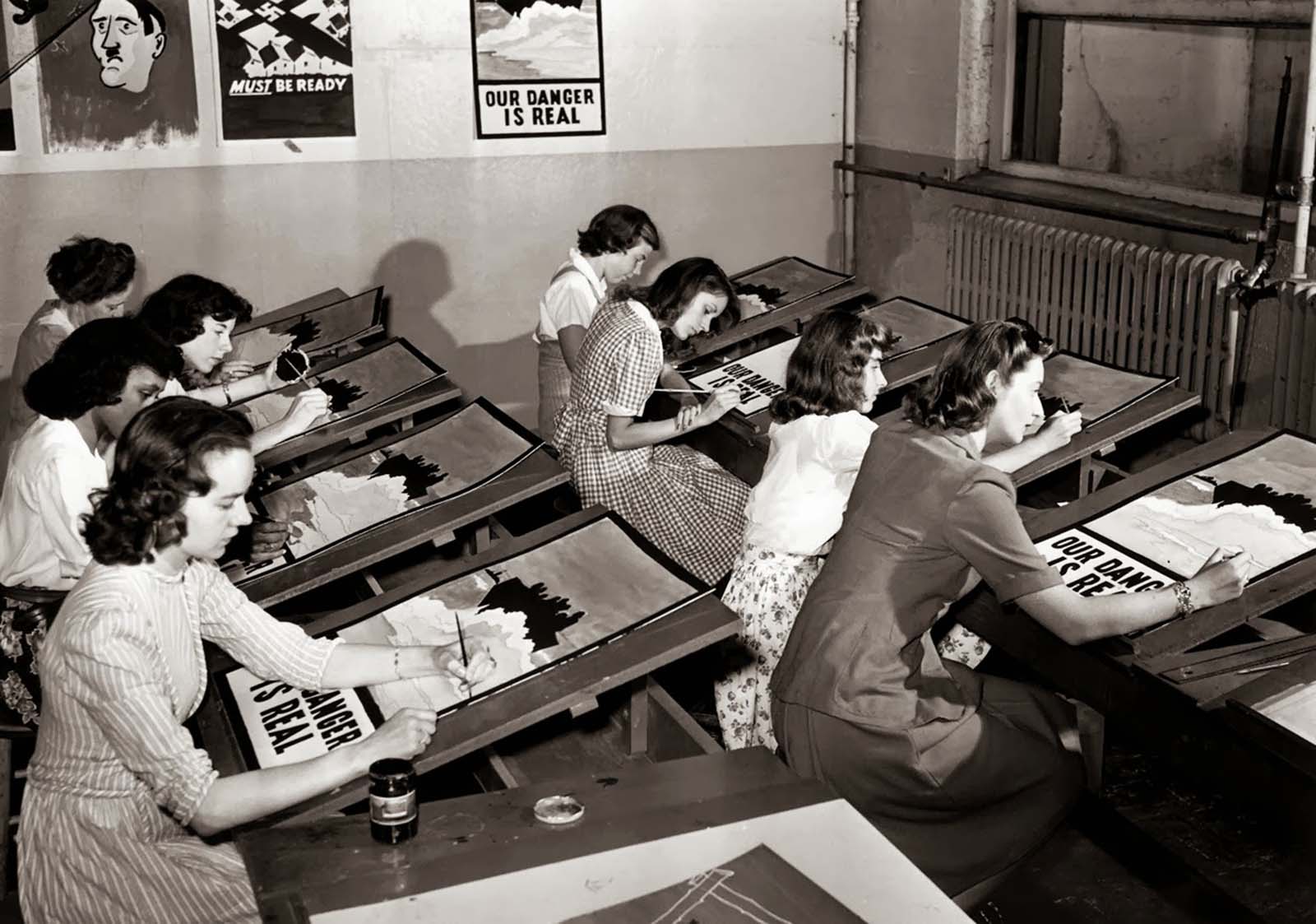The black-and-white photograph captures a detailed, intense scene inside a workshop corner where teenage girls are meticulously hand-coloring propaganda posters. Each girl is seated at an inclined drafting table, which is a flat brown wood panel, organized in two neat rows of workstations. The posters they are working on feature a rectangular design with bold text stating, "Our danger is real." The central image depicts a ship silhouette against white, cloud-like waves with another ship faintly visible in the far distance. On the wall behind them, additional propaganda posters are displayed, some with Nazi symbols and a cartoonish depiction of Adolf Hitler’s face. A heater is mounted on the far right wall, adding a touch of mundane reality to this eerie, highly controlled atmosphere. Overall, the photograph exudes a sense of uniformity and youthful labor dedicated to wartime propaganda efforts.